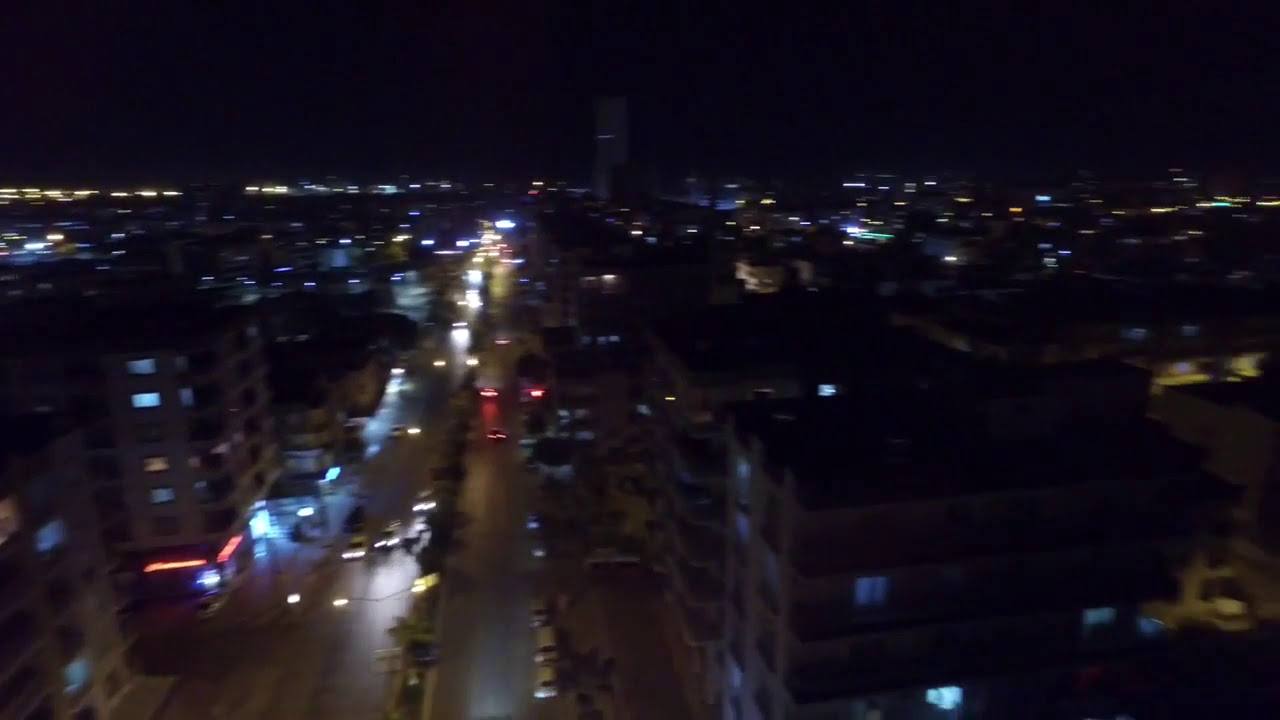This nighttime photo, taken from a high vantage point, captures a blurred yet bustling cityscape. The scene features lit buildings, with some windows illuminated and others dark, hinting at a mix of residential and office spaces. Below, a multi-laned street or highway stretches out, partially divided by tree-lined medians. On this road, traffic flows in opposite directions, evidenced by the glow of headlights coming towards the viewer and taillights heading away. The deep midnight blue sky forms the backdrop to this urban tableau, imbuing the image with an enigmatic nocturnal ambiance. The blur suggests motion, either from the person taking the photo or the vehicles themselves.